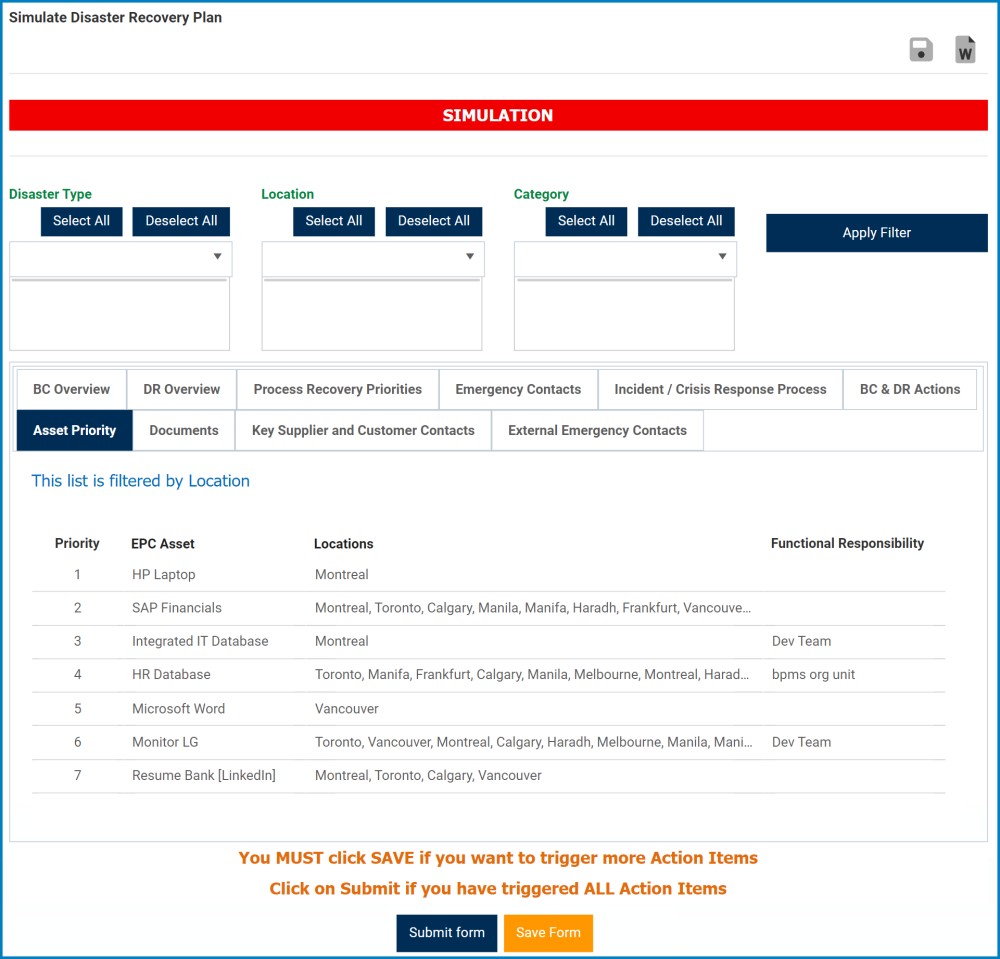**Detailed Caption:**

At the very top of the image, bold black letters on a white background read "Simulate Disaster Recovery Plan." Directly below this title, a prominent red rectangle is labeled "Simulation." Beneath this header, the layout is divided into clearly defined sections with the following details:

1. **Filters:**
   - The first section is titled "Disaster Type." Within this section, two black rectangles containing green text display the options to "Select All" and another option that is not fully visible.
   - The next section, labeled "Location," also includes two black rectangles with green text, offering the options to "Select All" and "Deselect All."
   - The third section, "Category," similar to the previous sections, contains black rectangles labeled "Select All" and "Deselect All."
   - At the bottom of these filter sections is a black rectangle marked "Apply Filter."

2. **Content Boxes:**
   - Below the filters, there are white rectangular boxes labeled as follows: "BC Overview," "DR Overview," "Process Recovery Priorities," "Emergency Contacts," and "Incident Crisis Response."

3. **Notice:**
   - Below the content boxes, it mentions, "This list is filtered by location," followed by a list labeled "EPC Access" and associated locations, along with a "Priority List."

4. **Action Buttons:**
   - At the bottom of the image, an orange text provides final instructions: "You must save. Click if you want to trigger more action items. Click on submit if you have triggered all action items."

This detailed caption encapsulates the intricate layout and specific instructions that guide users through the functions of a disaster recovery plan simulation interface.